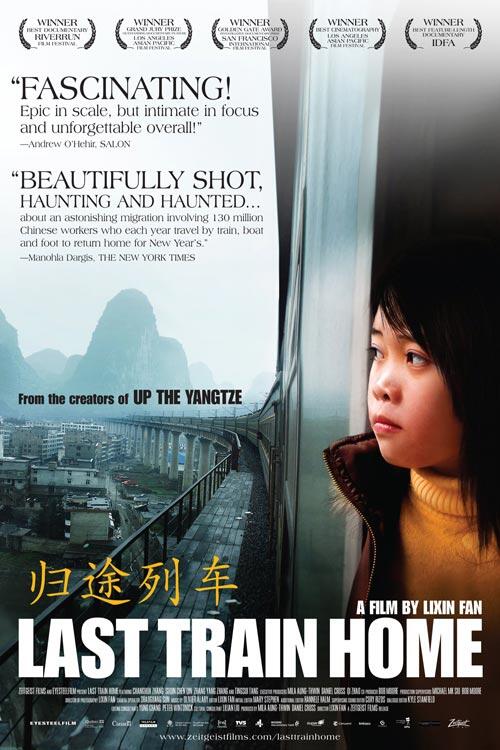The promotional poster for the movie "Last Train Home" features an evocative image of an Asian girl gazing out of the side of a train. The scene is set against a backdrop of a path with large stone steps, leading down to a city that can be seen below. This rectangular image, approximately six inches tall and three to four inches wide, is filled with intricate details.

At the very top, a central line of laurel leaves bear the word "Winner," signifying various accolades. Among them, the awards for Best Documentary, Grand Jury, and Best Cinematography are discernible. Beneath these laurels, a quote from Andrew O'Hare of Salon magazine praises the film as "fascinating epic in scale but intimate and focused and unforgettable overall." Another quote from Manohla Dargis of The New York Times describes the film as "beautifully shot, haunting and haunted," noting its depiction of "an astonishing migration involving 130 million Chinese workers who each year travel by train, boat, and foot to return home for New Year's."

Further down, the poster credits the creators, mentioning "from the creators of Up the Yanks." The title and creator of the film are displayed prominently at the bottom: "A film by Lixin Fan," titled "Last Train Home." Additionally, some Chinese script appears in yellow. This visually striking poster conveys the poignant story and intricate cinematography of the film.